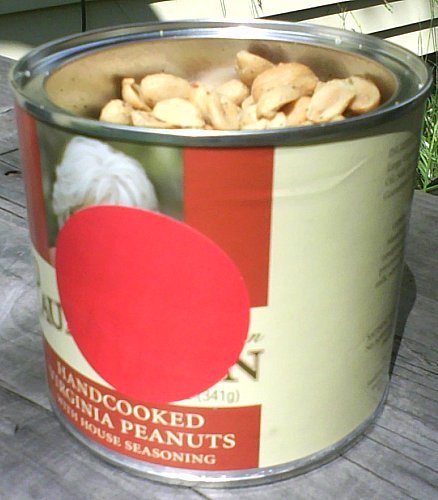This photograph depicts an open can of hand-cooked Virginia peanuts with house seasoning, prominently featuring a large red circular sticker that obscures much of the label. The can itself is off-white and burnt orange, with pale yellow lettering on a red background at the bottom indicating "hand-cooked Virginia peanuts with house seasoning." The silver rim of the open can reveals visible peanut halves inside. The label behind the sticker seems to have an image partially obscured, possibly of a woman with white or gray hair, suggesting it might depict Paula Deen. This container is placed outdoor on a weathered wood tabletop, with greenery faintly visible in the well-lit background. Additionally, the setting includes the side view of a shingled house, adding to the outdoor ambiance of the photograph.